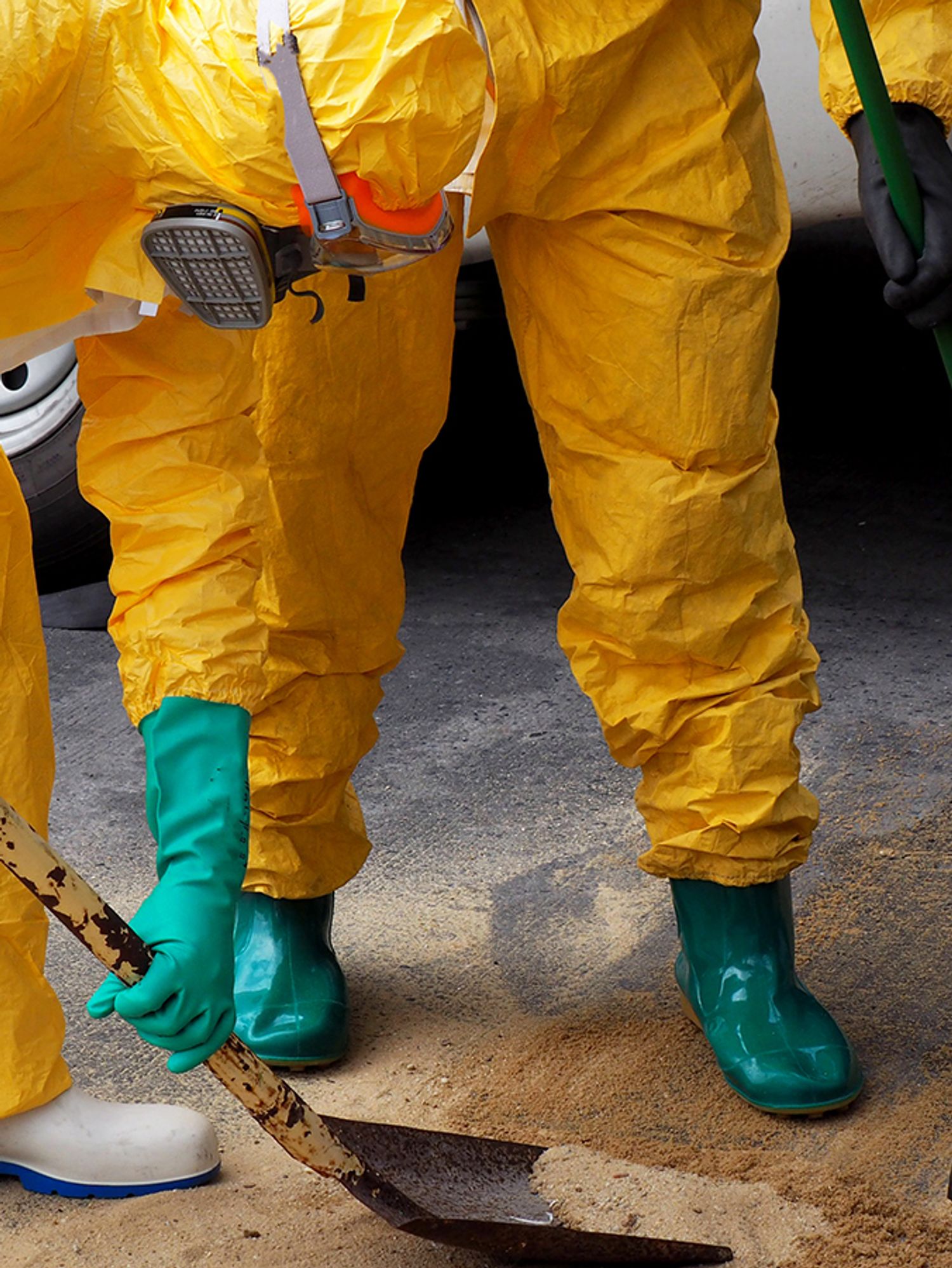In the photograph, two workers dressed in yellow protective hazmat suits are focused on their tasks on a gray, cemented ground scattered with tan sand mixed with black specks. The worker on the right, whose upper body is partially out of the frame, is identifiable by his black gloves and green boots. He appears to be holding a broomstick in his left hand. The worker on the left is bent over, actively shoveling the sand with a long-handled shovel that has a gray end and a yellow handle, which is worn and chipped. This worker is outfitted with a distinctive face mask featuring gray and red elements, paired with goggles that have an orange frame and a clear visor, secured by gray straps. He also wears long green gloves and blue and white boots. In the background, a white van with black tires and silver rims can be seen, adding context to their work environment.